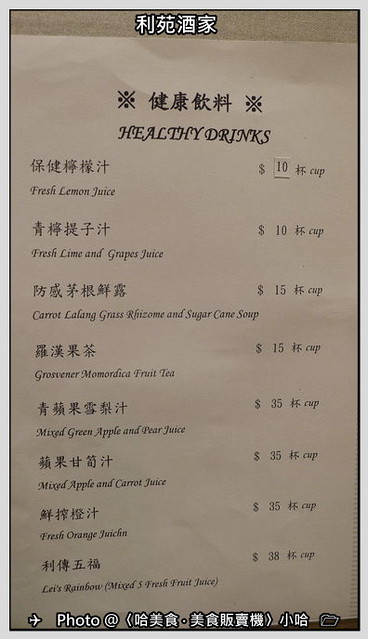A menu at a Chinese restaurant appears to be displayed on the wall, evidenced by visible tape at the top and a single glued-on price correction. The menu's header features a line of Chinese text accompanied by decorative icons resembling crosses with four dots. Immediately below, the header "Healthy Drinks" is presented in English. 

Each beverage listing begins with Chinese text followed by its English translation in italics:

1. Fresh Lemon Juice - $10 per cup
2. Fresh Lime and Grapes Juice - $10 per cup
3. Carrot, Lilang Grass Rhizome, and Sugar Cane Soup - $15 per cup
4. Gross Spinner Mordica Fruit Tea - $15 per cup
5. Mixed Green Apple and Pear Juice - $35 per cup
6. Mixed Apple and Carrot Juice - $35 per cup
7. Fresh Orange Juichen (noted typo for Juice) - $35 per cup
8. Lay's Rainbow Mixed Five Fresh Fruit Juice - $38 per cup

At the bottom of the image, white Chinese text is accompanied by an airplane icon and a folder icon, possibly indicating that the picture was taken with a cell phone and what we see is the phone's viewfinder. The presence of a gray border initially suggested a frame, but it might be part of the phone's interface, adding some ambiguity about the exact presentation of the menu.